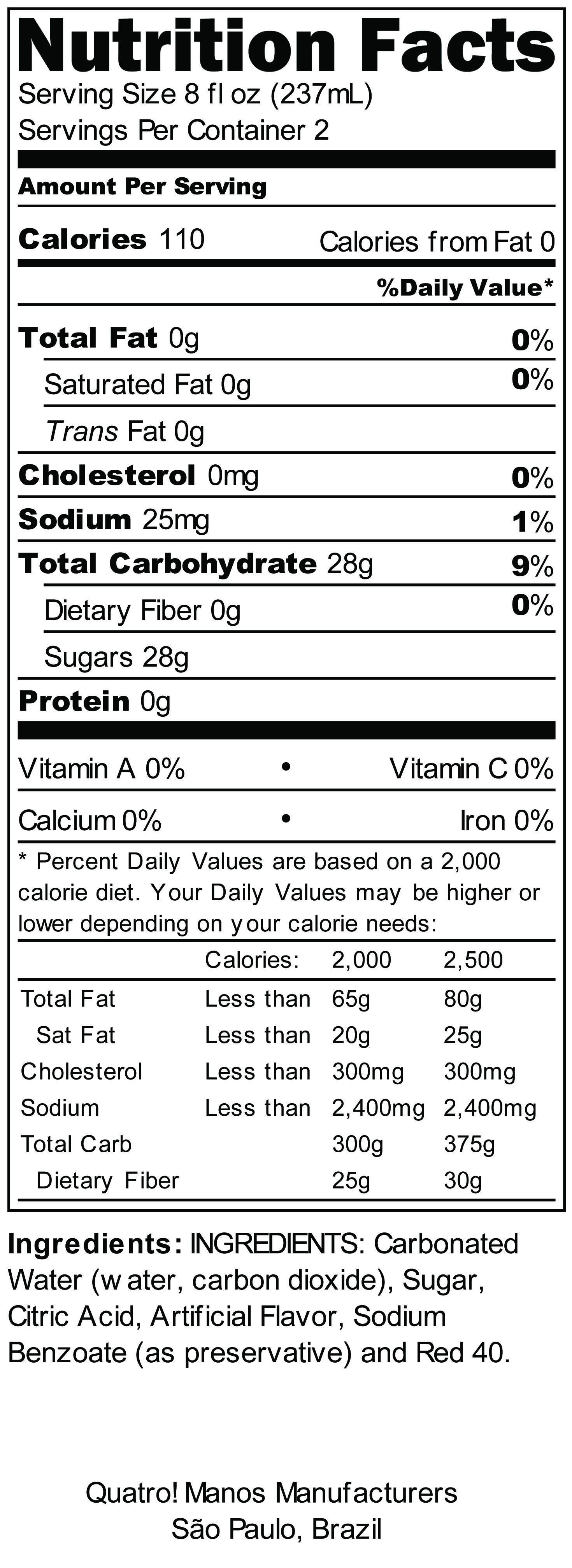This image showcases the nutritional information and ingredient list from a typical store-bought beverage. The nutrition facts panel indicates that the serving size is 8 fluid ounces and the container holds 2 servings, making a total of 16 fluid ounces. Each serving provides 110 calories, with no calories from fat. The beverage contains no cholesterol and a minimal amount of sodium, accounting for 1% of the daily recommended intake. It provides 28 grams of total carbohydrates per serving, which is 9% of the daily value, all of which comes from sugars, amounting to 28 grams. The drink offers no protein, vitamin A, vitamin C, calcium, or iron.

The ingredient list includes carbonated water, sugar, citric acid, and artificial flavor. Sodium benzoate is used as a preservative, and the beverage is colored with Red 40. This product was manufactured in São Paulo, Brazil.